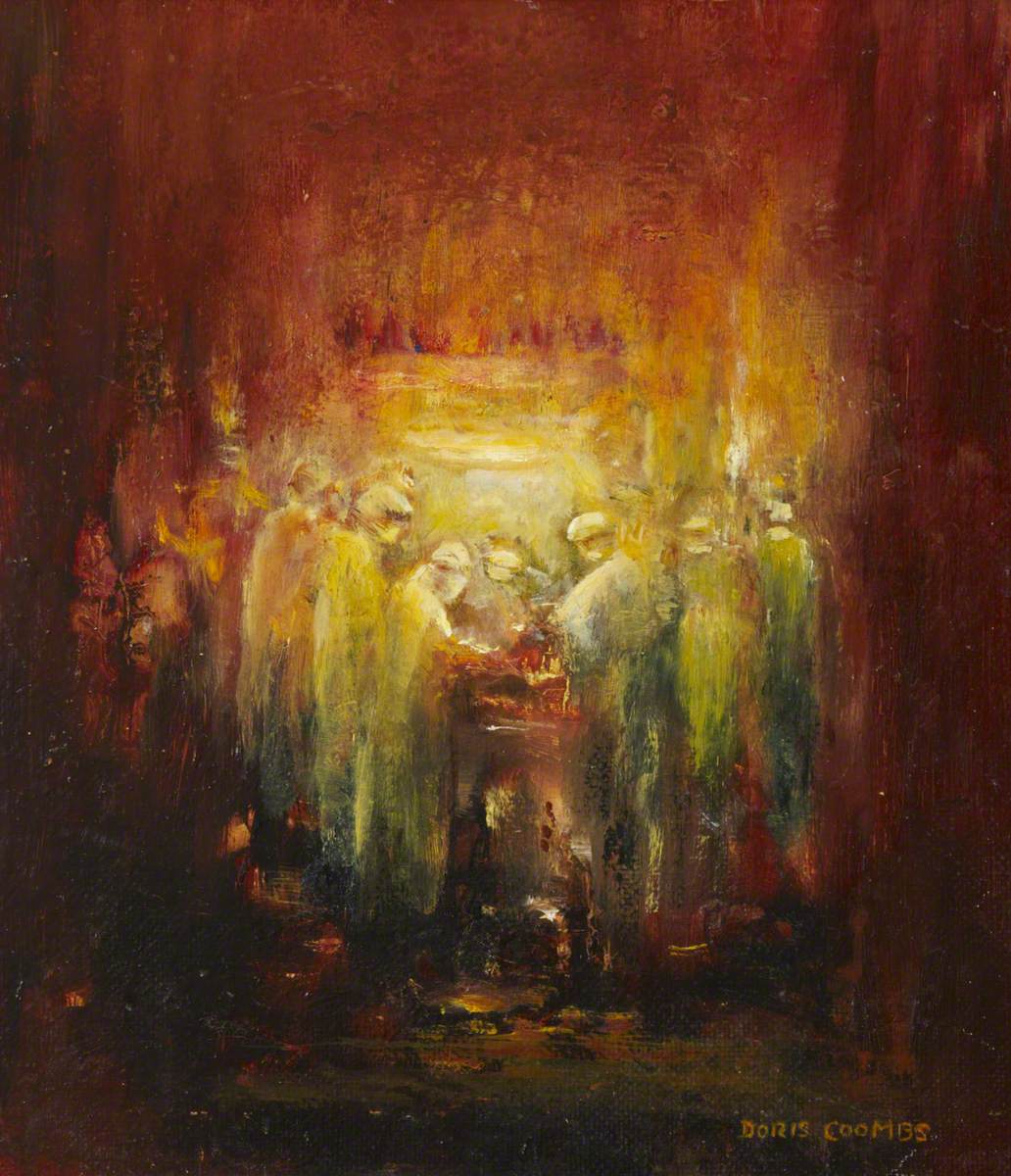This is an oil painting by Doris Coombs, signed in the bottom right corner. The artwork, done in a modern impressionistic style, primarily features rich earthy tones of burnt umber and dark reds, which gradually shift to bright yellows and whites towards the center. The composition encircles an operating table, emphasizing an impression of a surgical scene. The painting portrays an indistinct yet evocative assembly of doctors in surgical gowns, face masks, and head coverings, appearing almost ghostly due to the low-detail impressionistic technique. Approximately ten surgeons are gathered around the table, their forms blending seamlessly with the background, suggesting the intensity and unity of their task. The painting also includes subtle hints of greenish-blue within its rich, airbrushed textures.